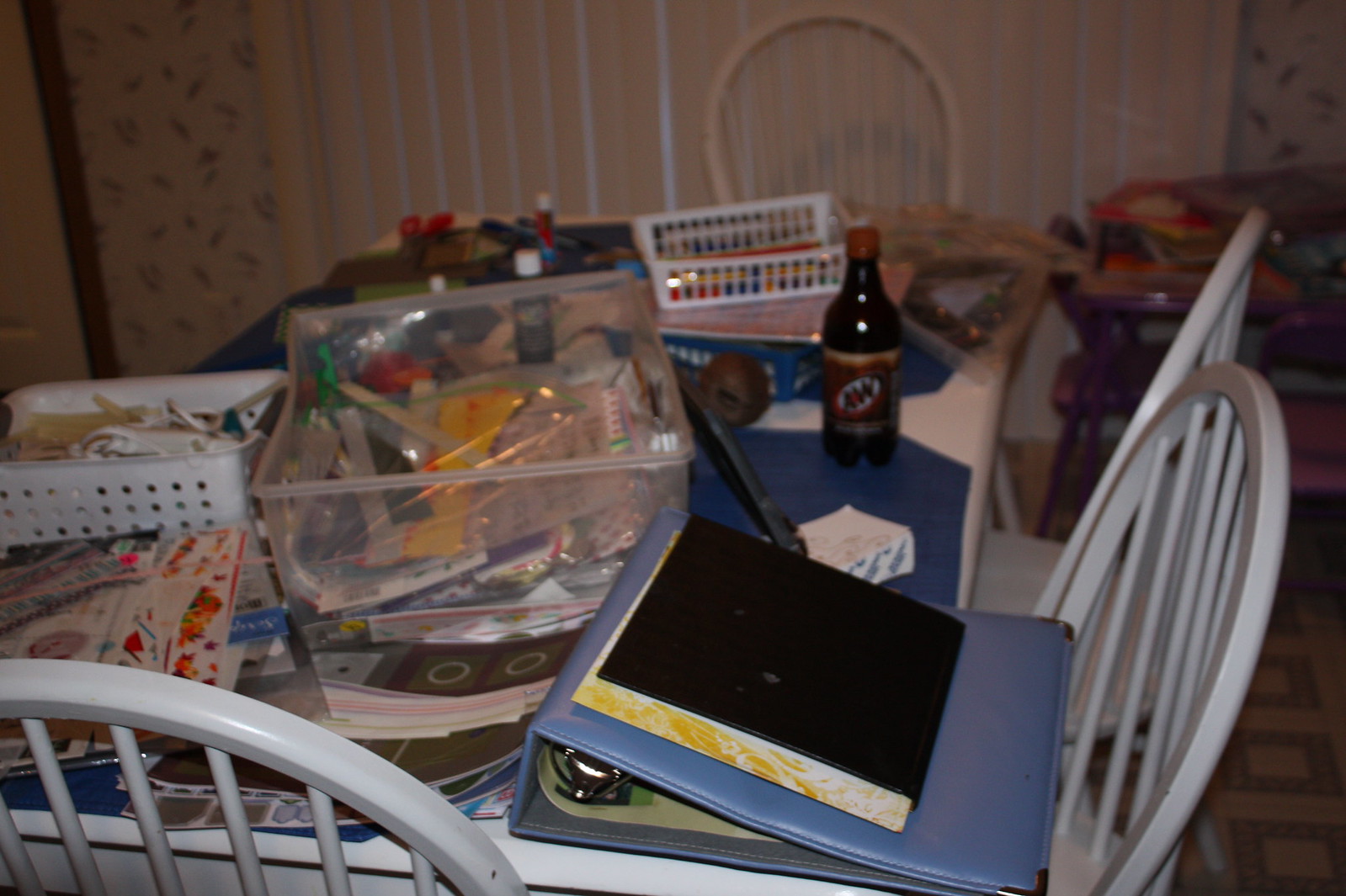This landscape-oriented image captures the chaotic scene of someone's kitchen illuminated by a camera flash. The focal point is a long wooden table at the center, surrounded by four white wooden chairs. The table is cluttered with an assortment of items including notebooks, binders, various craft supplies, and magazines strewn about haphazardly. Notable objects include a plastic A&W Root Beer bottle positioned towards the right side and several pens scattered across the surface. The table also features multiple bins filled with office supplies; one is see-through, while others are white and contain various materials. On the left side of the table, an untidy stack of magazines contributes to the overall disorganized appearance of the space. This image vividly depicts a messy, lived-in kitchen environment.